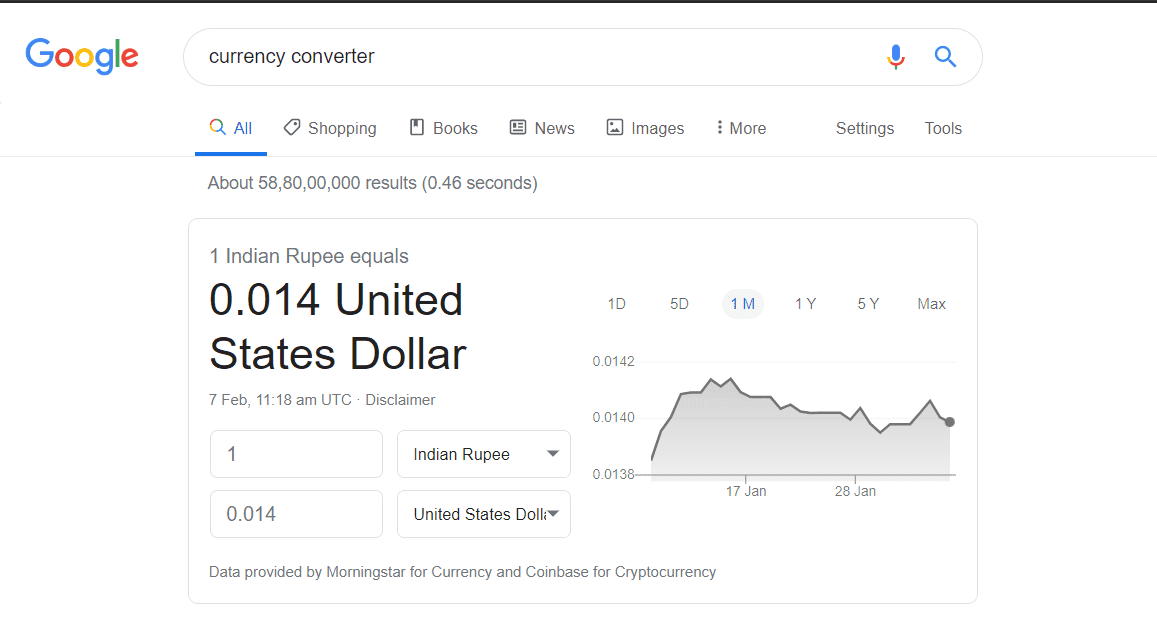This image displays a Google page with the heading "Currency Converter," presenting the conversion rate between Indian rupees (INR) and United States dollars (USD). On February 7th at 11:18 AM UTC, the exchange rate was 1 Indian Rupee (INR) to 0.014 United States Dollars (USD). The data for this conversion is sourced from Morningstar for currency and Coinbase for cryptocurrency. At the bottom of the page, a graph tracks the exchange rate fluctuations between January 17th and January 28th, illustrating a downward trend in the value of the Indian Rupee during this period. The page also contains additional, unspecified figures.